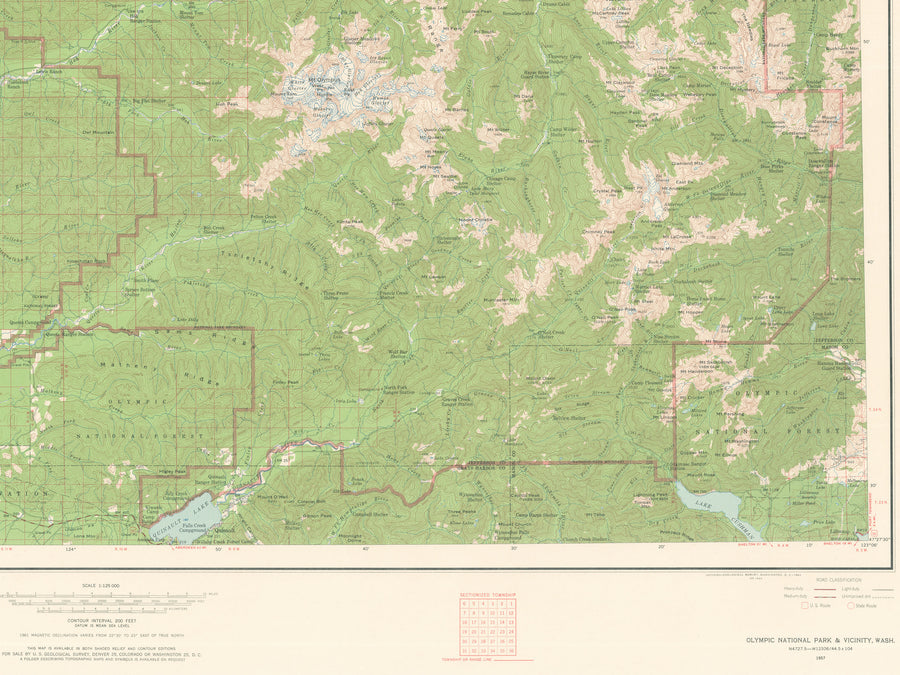The image depicts a top-down view of a detailed map, whose specific location is unclear. The map prominently features green terrain with patches of light tan or beige, possibly indicating varying elevations or land types. Thin, light brown lines form a rectangular grid crisscrossing the map horizontally and vertically, with thicker lines delineating distinct areas or boundaries. Toward the bottom of the map, there are two bluish regions, likely representing bodies of water, positioned on the left and right sides. Below the map itself, a white section contains small, difficult-to-read text. In the bottom-left corner of this section, there's some writing, and in the bottom-right corner, the text "Olympic National Park and vicinity, Wash." can be seen. A red box with indistinguishable numbers is centered at the bottom of the map.